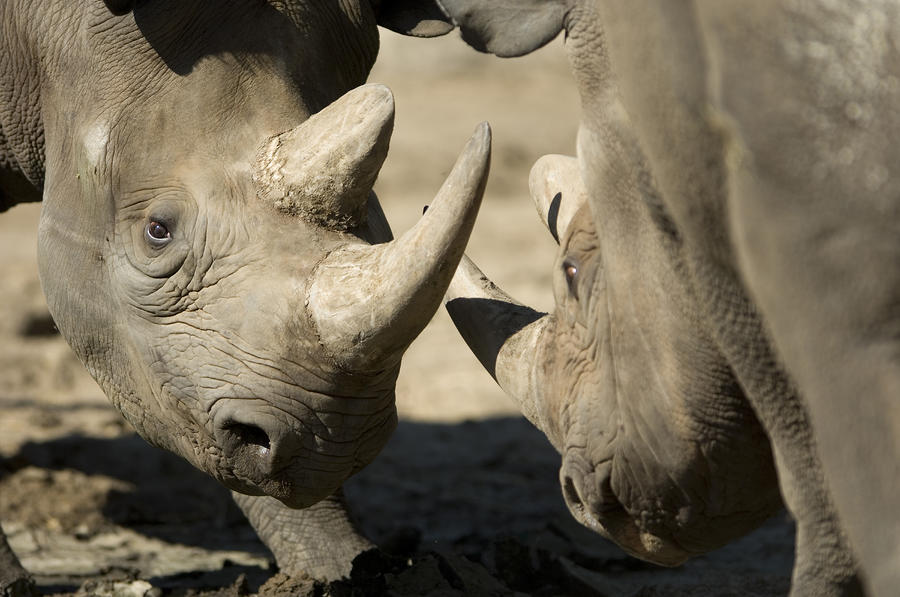In this crystal-clear photograph, two dark gray rhinoceroses are captured in a seemingly tense moment, poised as if about to spar. The ground beneath them is brown, potentially muddy, with the sun shining brightly in the background casting their silhouettes into sharp relief. The rhinoceros on the left is more clearly visible, with its face, part of its leg, and its neck in focus, showcasing its big brown eyes, large nostrils, and two impressive horns; the shorter horn is accompanied by a taller, sharper one that looks formidable. The rhinoceros on the right, although slightly blurred, reveals part of its head and body, also featuring a pair of horns. Both animals have leathery, wrinkled skin and are positioned with their heads down close to the ground, their horns nearly touching, suggesting an imminent confrontation.